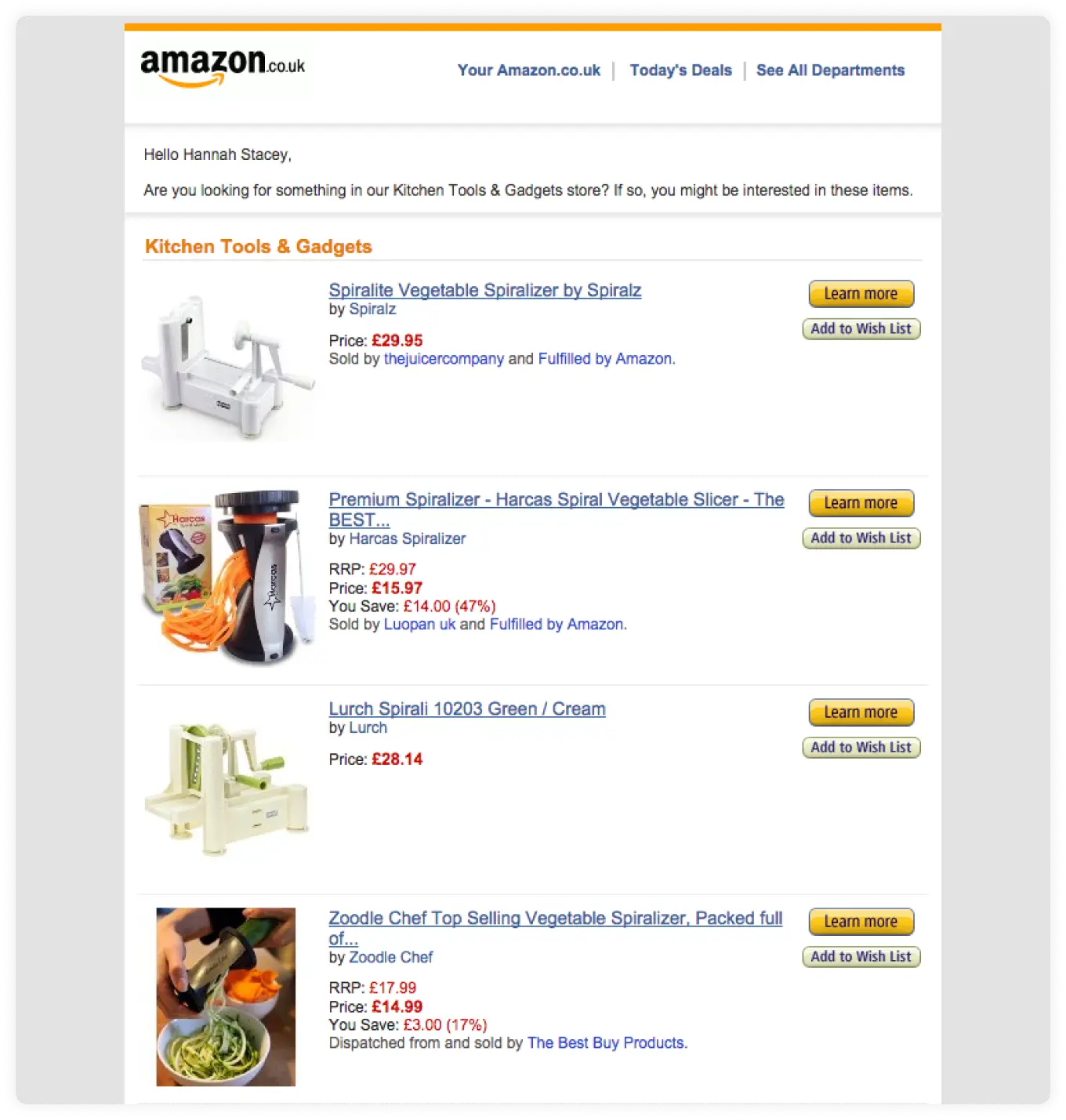**Descriptive Caption for the Image:**

This is a screen capture from the Amazon.co.uk website, depicting a product recommendation page. The image features a predominantly white background overlaid on a gray backdrop. At the top of the image, a thin gold strip is visible, followed by the Amazon.co.uk logo, which includes the iconic gold swoosh between the 'A' and the 'Z'. Just below the logo, in blue, it reads: "Your Amazon.co.uk," "Today's Deals," and "CL Departments."

The text, displayed in black, greets the user: "Hello Hannah Stacey, are you looking for something in our kitchen tools and gadgets store? If so, you might be interested in these items." Below this greeting, there are four detailed product listings under the orange header: "Kitchen Tools and Gadgets."

1. **Product 1:** 
   - **Image:** Depicts the Sperlet Vegetable Spiralizer by Spirals.
   - **Price:** £29.95 
   - **Sold By:** The Juice Juicer Company and fulfilled by Amazon.
   - **Buttons:** Learn More and Add to Wishlist.

2. **Product 2:** 
   - **Image:** A silver and black spiralizer device next to its box.
   - **Description:** Harkis Spiral Vegetable Slicer, the best by Harkis Spiceler.
   - **RRP:** £29.97 
   - **Price:** £15.97 
   - **Savings:** Save £14 or 47%.
   - **Sold By:** Leucopan UK and fulfilled by Amazon.
   - **Buttons:** Learn More and Add to Wishlist.

3. **Product 3:** 
   - **Image:** A green and white spiralizer device.
   - **Description:** Lurch Spiral 10203 Green and Cream by Lurch.
   - **Price:** £28.14
   - **Buttons:** Learn More and Add to Wishlist.

4. **Product 4:** 
   - **Image:** Shows a lighter-skinned person using a silver and green spiralizer, with two white bowls containing sliced items nearby.
   - **Description:** Zoodle Chef Top Selling Vegetable Spiralizer.
   - **RRP:** £17.99
   - **Price:** £14.99
   - **Savings:** Save £3 or 17%.
   - **Sold By:** The Best By Products.
   - **Buttons:** Learn More and Add to Wishlist. 

The image showcases these recommended kitchen tools and gadgets, providing pricing, seller information, and interactive buttons for further engagement.